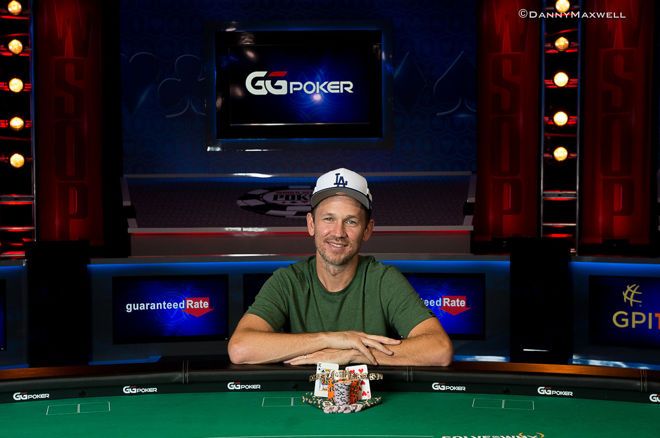The image captures a scene inside a poker room featuring a man seated at a green poker table. The table, lined with white markings and bordered by a black edge, displays a spread of poker cards and a stack of black and white poker chips in front of the man. Notably, a King of Spades is positioned to the left, and a pair of Sevens of Hearts is on the right. The man, who sports a bit of facial hair, wears a white baseball cap with "L.A." emblazoned on it and a green T-shirt. His hands rest on the black edge of the table, with his left arm underneath his right and fingers touching his forearm. He has a slight smile, revealing some teeth and adding a sparkle to his eyes. The background includes a TV screen displaying "GG Poker" alongside various colored neon lights and additional advertisements, such as "Guaranteed Rate." The overall ambiance suggests a professional poker setting, capturing the player's poised yet approachable demeanor.